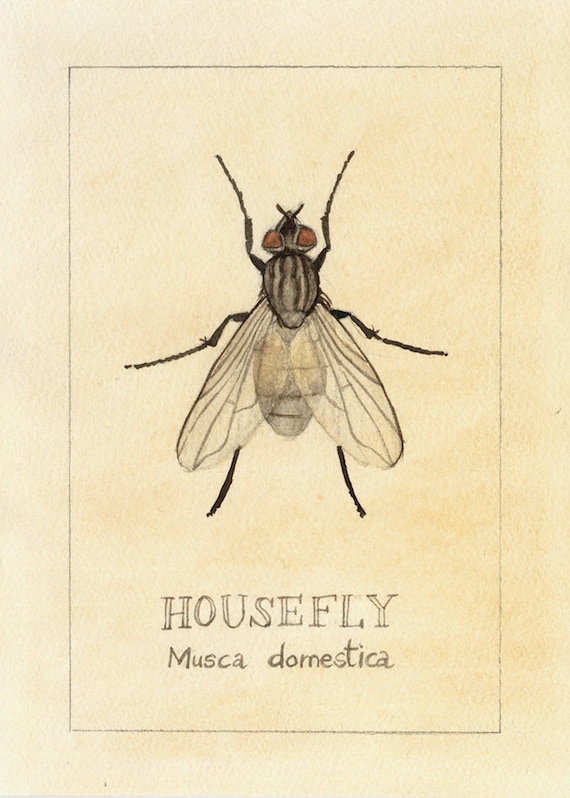The image depicts a detailed illustration of a housefly, centrally positioned on a faded, ivory-colored background, resembling aged paper with a peach and cream tint. The fly's body features a mix of black and gray with discernible black stripes. It has six black legs and two antennae. The fly's eyes are a striking reddish-orange, and its sheer, creamy wings are notably transparent. Below the image, the words "House Fly" and "Musca domestica" are prominently displayed in black letters. The entire image is framed by a black border, suggesting it might be an art piece suitable for wall display.